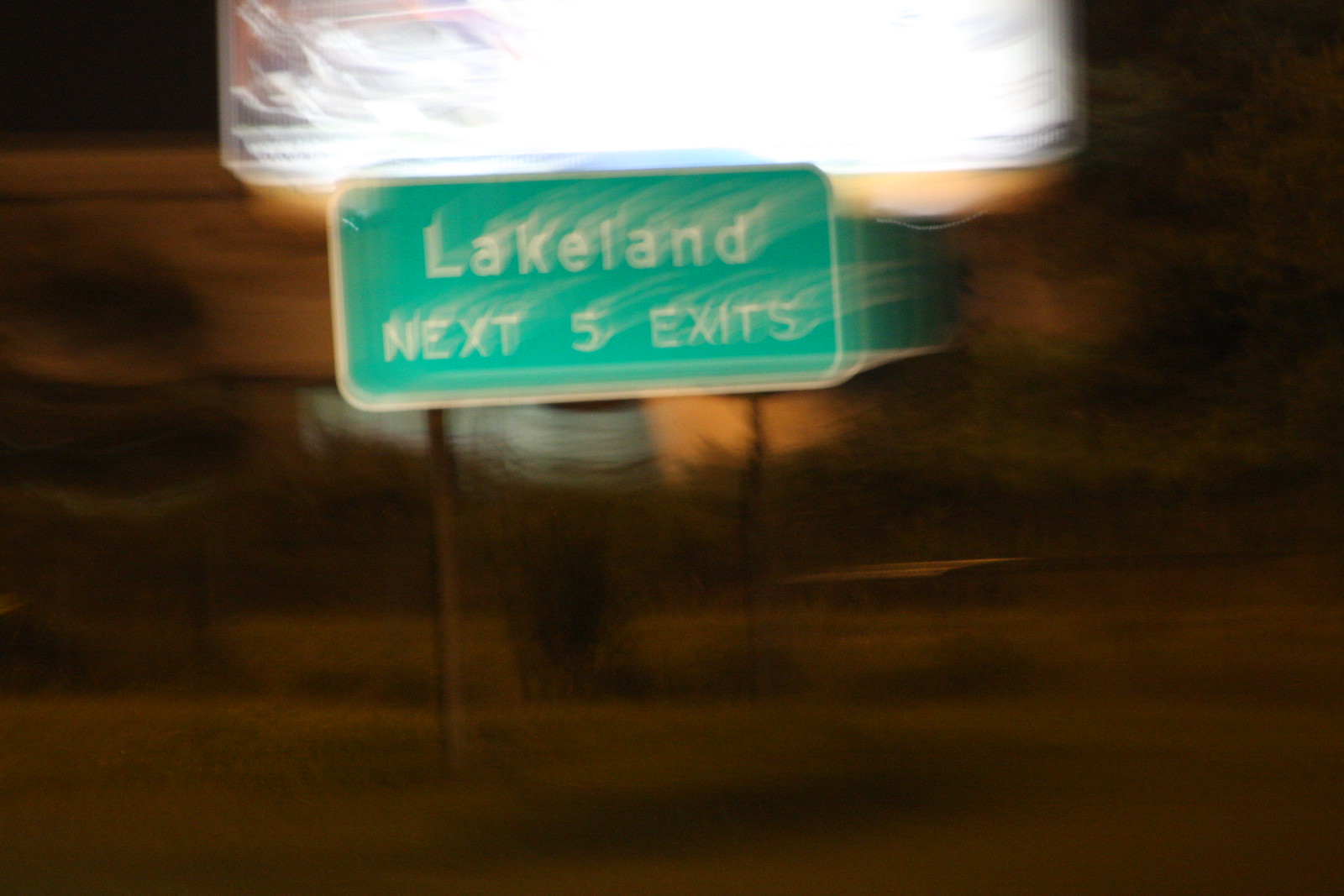A nighttime photograph, captured from a moving car, shows a blurry landscape with patches of grass, bushes, and scattered shrubs. Dominating the scene is a green highway sign on a metal pole, labeled "Lakeland" in white letters, with an indication for the "next five exits" beneath it. Adjacent to this sign is an elevated and brightly illuminated billboard, though its message is indistinguishable due to the image's blurriness. The remaining background fades into darkness, with the flat landscape just barely visible below the sign and billboard.